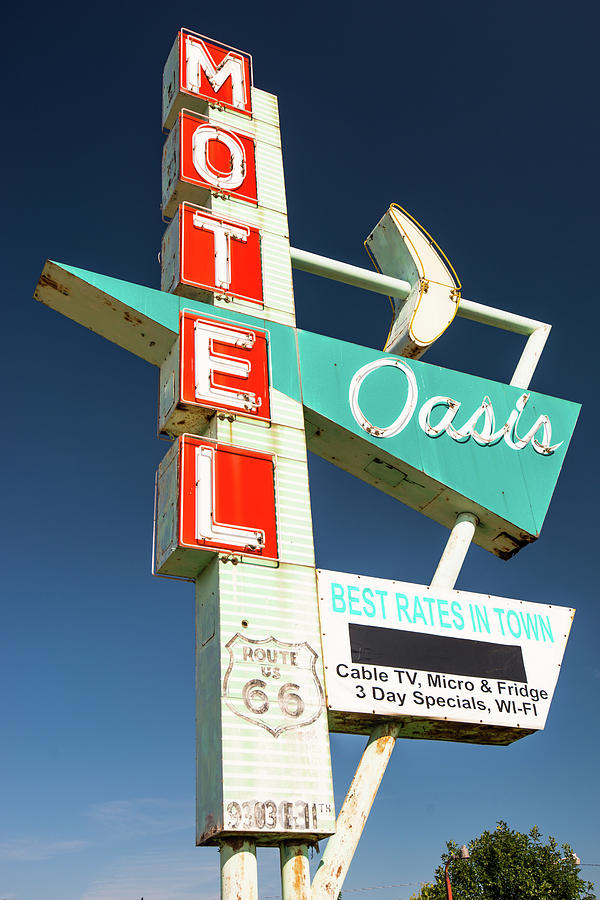The image features a towering motel sign set against a clear blue sky. The sign is vertically oriented, with the word "MOTEL" prominently displayed in white letters on individual red blocks that descend from top to bottom. To the right of these blocks is a turquoise triangle with the word "Oasis" elegantly scripted in white font. Below this, in the lower right corner, several smaller shapes contain various bits of information: "Best Rates in Town" in blue font, and beneath it, in black font, details such as "Cable TV," "Micro and Fridge," "Three Day Specials," and "Wi-Fi." The sign also features "Route 66," evoking nostalgic Americana from the 1950s or early 60s, accentuated by its slightly rusted metal frame. In the background, a verdant tree and a streetlight are visible, further grounding the scene in an outdoor, sunny atmosphere.